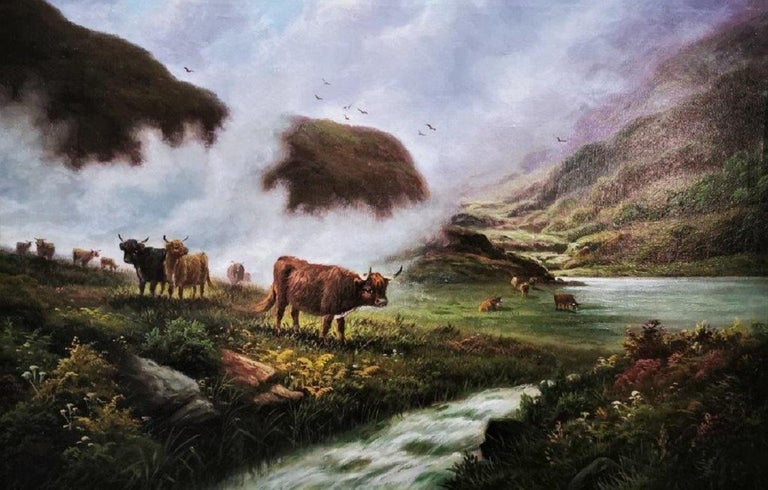This painting depicts a misty valley scene centered around a herd of wild, long-furred cattle grazing and resting near a delicate, fast-flowing stream. The cattle, mostly brown with some darker and scrubby, prominent long-horned breeds, are dispersed across a riverbank lush with green grasses and vegetation. A notable black cow stands out amidst them, positioned near the center, walking with its head to the right and tail to the left. The backdrop features an imposing, mist-covered mountain that extends high into the sky, partially obscured by the fog. Above, a dynamic sky filled with heavy, puffy purple clouds and dark-colored birds adds to the dramatic atmosphere of the scene, with the sunlight casting illumination on various parts of the landscape, enhancing the serene yet wild beauty of the valley.